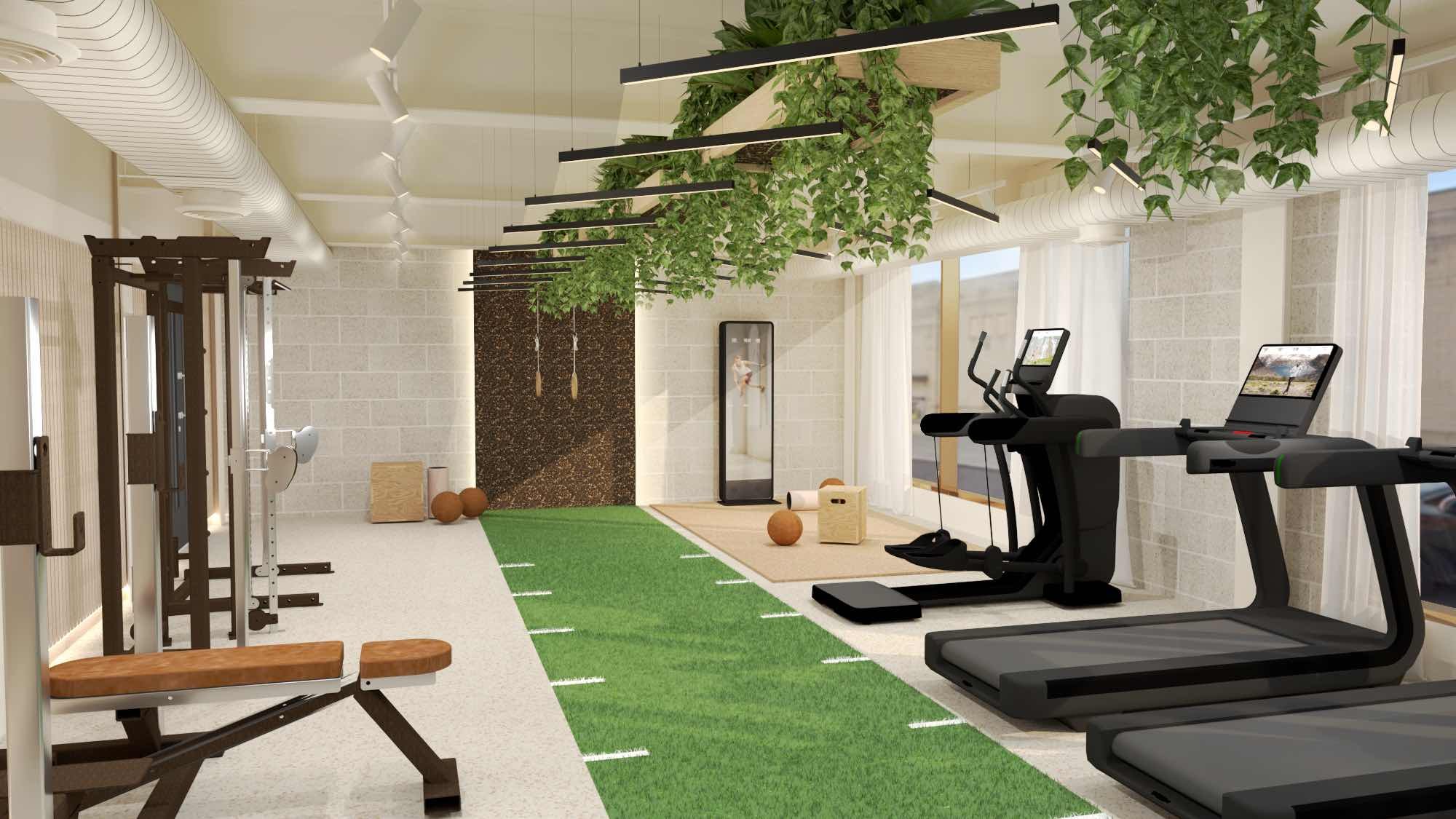This is an image of a modern indoor exercise room with cinderblock walls that have a gray color with white borders. Along the ceiling, plants with green vines are suspended in boxes, stretching from one end of the room to the other, and interspersed with light fixtures. Underneath the greenery is a central patch of artificial turf that resembles a football field, complete with white lines on the sides, and terminates at a brownish wall. Towards the lower and center right of the room, there are several treadmills and an elliptical machine, each equipped with large monitor screens likely used for virtual coaching. Adjacent to these machines, slightly further back, is additional workout equipment. On the left side of the photograph, weightlifting gear is arranged below a white ventilation duct with several outlets. Basketballs are visible in the background near a dark brown door. The overall ambiance is enhanced by the hanging plants, creating an inviting and vibrant exercise environment.